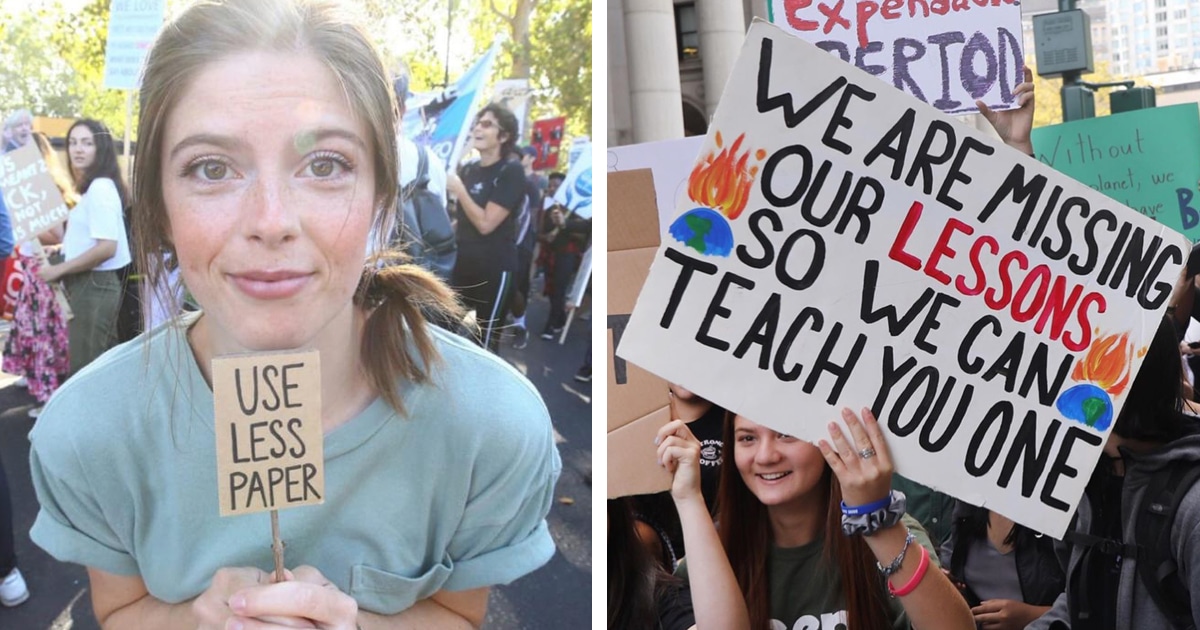This image features two photographs placed side-by-side, each capturing a moment from a protest. On the left is a detailed shot of a woman with loosely pulled-back brown hair, draped over her left shoulder. She wears a blue t-shirt with rolled-up sleeves and is gazing directly into the camera, her face adorned with mascara and lipstick. In her hands, she holds a small sign attached to a block of wood, bearing the message "Use less paper" written in black marker. The background reveals a bustling protest scene with various demonstrators and their signs visible under the sunlight that suggests early daytime.

To the right, another young woman is prominently featured, holding a large poster board that dominates the frame. Her long brown hair cascades down her green t-shirt, which is decorated with white writing. She wears numerous bracelets on her wrists. The sign she holds commands attention with its bold black letters and red text, stating, "We are missing our lessons so we can teach you one," flanked by illustrations of the Earth topped with flames. Behind her, more protestors and their unreadable signs are visible against a backdrop of buildings and hints of daytime light.